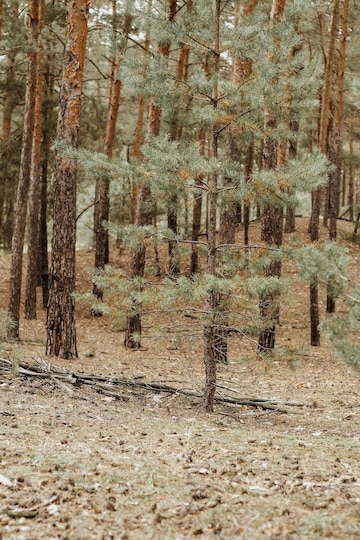This photograph captures a well-maintained young pine forest, likely around 6 to 8 years old, with a dense but navigable arrangement of vertical pine trees centrally positioned within the frame. The ground is scattered with light brown to gray twigs, pine needles, and pine cones, creating a natural carpet over the dirt. There are patches of grass and minimal brush, making it easy to move through the forest. The tree trunks are predominantly brown, with green pine leaves visible higher up on some trees, though the lower sections are mostly bare. Overall, the scene reflects the early growth stages typical of forests near paper mills, where trees are routinely harvested and replanted, allowing for clear pathways between them and a relatively clean forest floor.